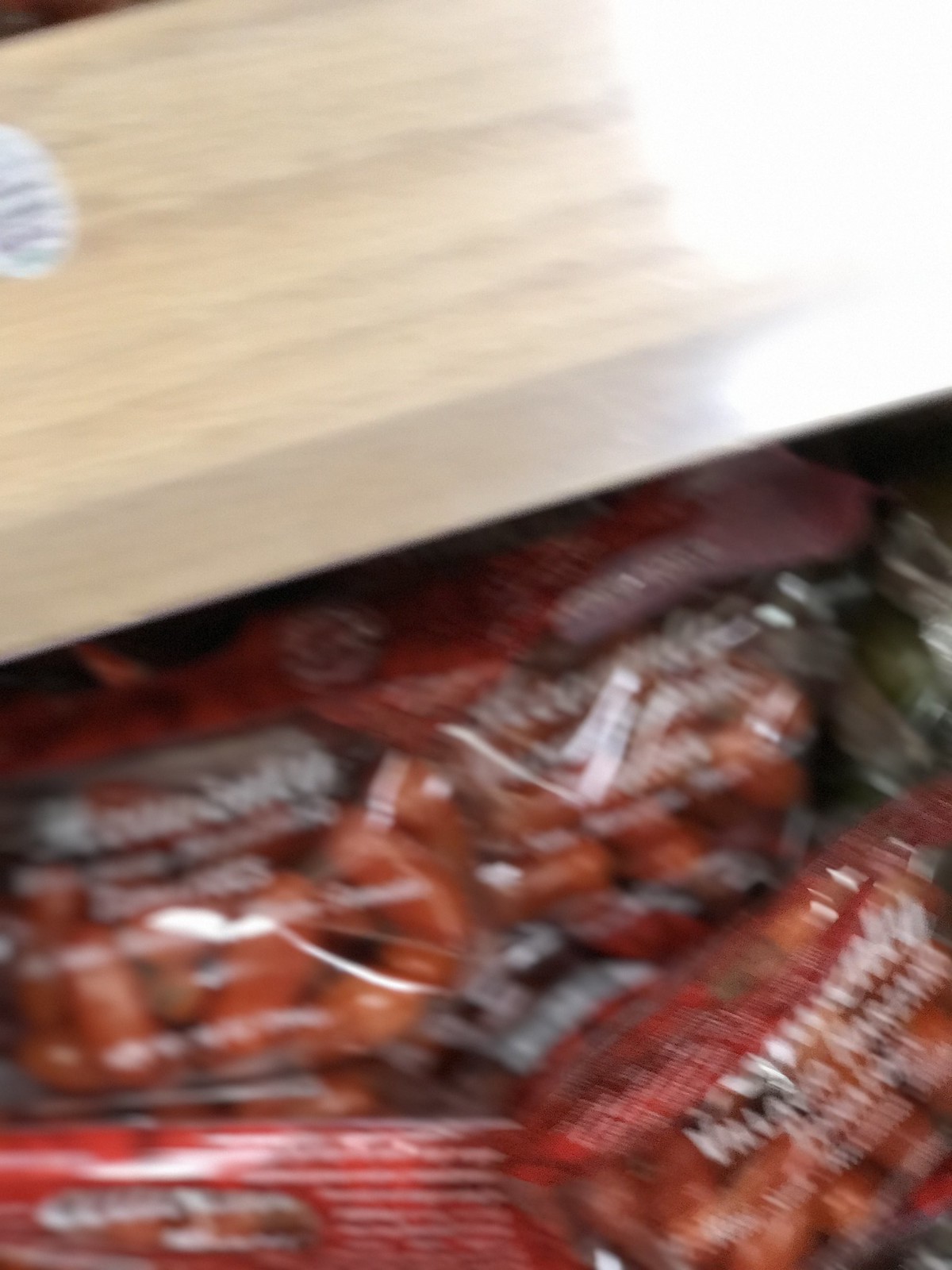In this indoor image, a brown laminate countertop is prominently featured. Below the countertop, there are stacks of plastic-wrapped items, characterized by vibrant red packaging with white text and reflections. The designs on the packaging suggest these items are likely sausages. The image appears to be taken near a freezer, contributing to the overall blur. A bright light in the top right corner reflects off the plastic packaging, further highlighting the items in focus.